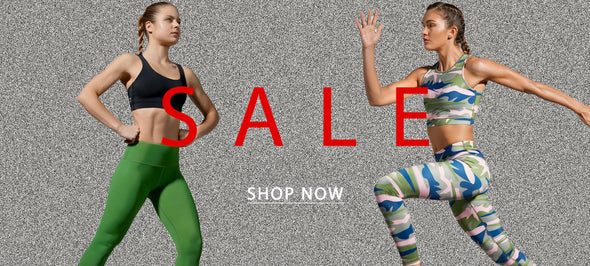The image features a landscape layout with a static-like, gray background composed of various shades of gray, black, and hints of blue. Centered on this backdrop are two athletic Caucasian women, both with their blonde hair pulled back in braids. The woman on the left is posed with her hands on her hips and wearing a black sports bra and tight green leggings, which reveal her muscular physique. Her head is slightly drooped, showing off a long ponytail flowing down her back. The woman on the right, also clad in a sports bra, is in a running stance, with her right hand in front of her face and her left arm extended behind her. She sports camouflage-patterned leggings and a matching sports bra in hues of white, blue, and green. Overlaying both women in bold red capital letters is the word "SALE", with "SHOP NOW" in smaller white capital letters below, underlined for emphasis. Both women are shown from just above the knees up, and their fit, toned bodies highlight the activewear being promoted.